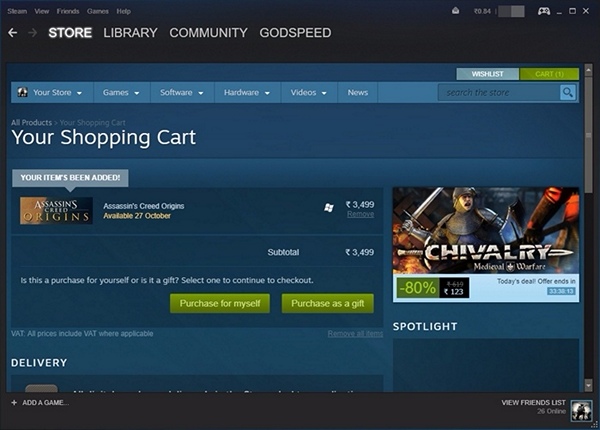This image is a detailed screenshot from an unidentified website, most likely an online gaming store, displaying various navigation options and shopping cart details. At the top of the page, there are tabs labeled "Store," "Library," "Community," "Godspeed," "Your Store," "Games," "Software," "Hardware," "Videos," "News," "Wishlist," "Cart," and a search bar labeled "Search the Store."

Prominently, there is a shopping cart section indicating that the game "Assassin's Creed Origins" has been added to the cart. The game is priced at 3,499 rupees and is set to be released on 27 October. Options are provided to either remove the item or proceed to checkout, with choices to purchase the game for oneself or as a gift. The subtotal is listed as 3,499 rupees, including VAT where applicable.

On the right side of the image, there's an advertisement featuring a knight in armor holding up a sword, promoting "Chivalry: Medieval Warfare" at an 80% discount for 123 rupees. This is noted as today's deal, with the offer ending in 33:38:13.

Additional elements on the page include options such as "Spotlight" and "View Friends List." The image notably lacks any photographic elements, animals, birds, plants, flowers, trees, or automobiles.